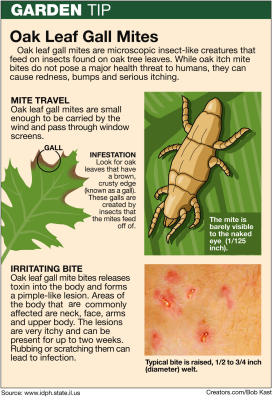The image depicts an informational poster titled "Garden Tip." At the top, there is a dark green header adorned with bold white block letters spelling "Garden" and thinner white letters reading "Tip." Below this header is a white section featuring the main heading in large black letters: "Oak Leaf Gall Mites."

The background of the poster is predominantly white, filled with detailed black text. The text begins by describing oak leaf gall mites as microscopic, insect-like creatures that inhabit and feed on insects found on oak tree leaves. It notes that while bites from these mites do not present severe health risks, they can cause redness, bumps, and intense itching.

On the left side of the poster, there are multiple sections of text labeled "Mite Travel," "Infestation," and "Irritating Bite." There is also an image of an oak leaf with pointed lobes typical of a black oak. The leaf is depicted with red edges, and a circled area labeled "Gall" highlights where the mites affect the leaf.

To the right, there is an illustration of the oak leaf gall mite, depicted as a pale beige insect with segmented body parts and eight legs, comprising sets of antenna-like forelegs, middle-section legs, and rear legs. Below this illustration, there is a photograph showing human skin with characteristic mite bites, appearing as red welts measuring approximately half to three-quarters of an inch in diameter.

Overall, the poster serves as a detailed resource on identifying and understanding oak leaf gall mites, their impact on oak trees, and the effects of their bites on human skin.